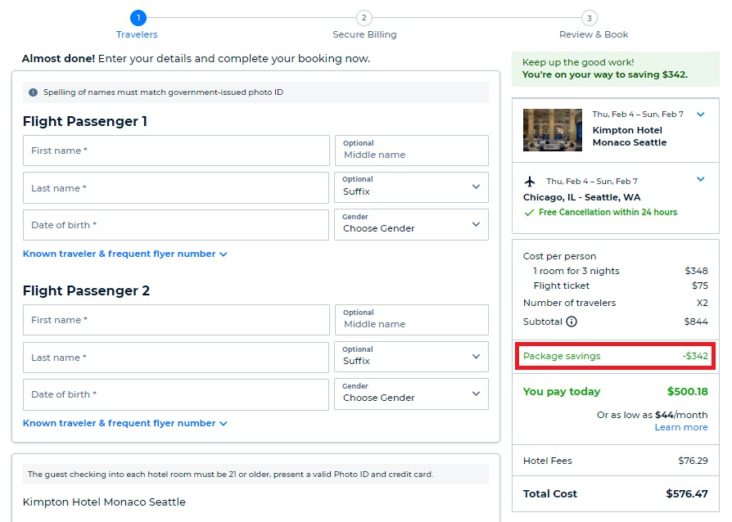In the image, travelers are engaged in the flight booking process on a digital booking page. The interface instructs users to secure billing, review, and finalize their bookings. The current stage is focused on the travelers' information.

Under the traveler details section, the page prompts users to enter accurate information, emphasizing that the spelling of names must exactly match those on government-issued photo IDs. The details for Flight Passenger 1 are empty, requiring inputs for first name, last name, and date of birth, along with fields for a known traveler number and frequent flier number. Similarly, Flight Passenger 2 also has empty fields for first name, last name, and date of birth, as well as sections for a known traveler number and frequent flier number.

Additional instructions highlight that the guest checking into each hotel room must be 21 years of age or older and must present a valid photo ID and credit card upon arrival. The accommodation mentioned is the Kimpton Hotel Monaco in Seattle. A confirmation message encourages users by noting they are on their way to saving $342 on their booking, from Thursday, February 4th to Sunday, February 7th.